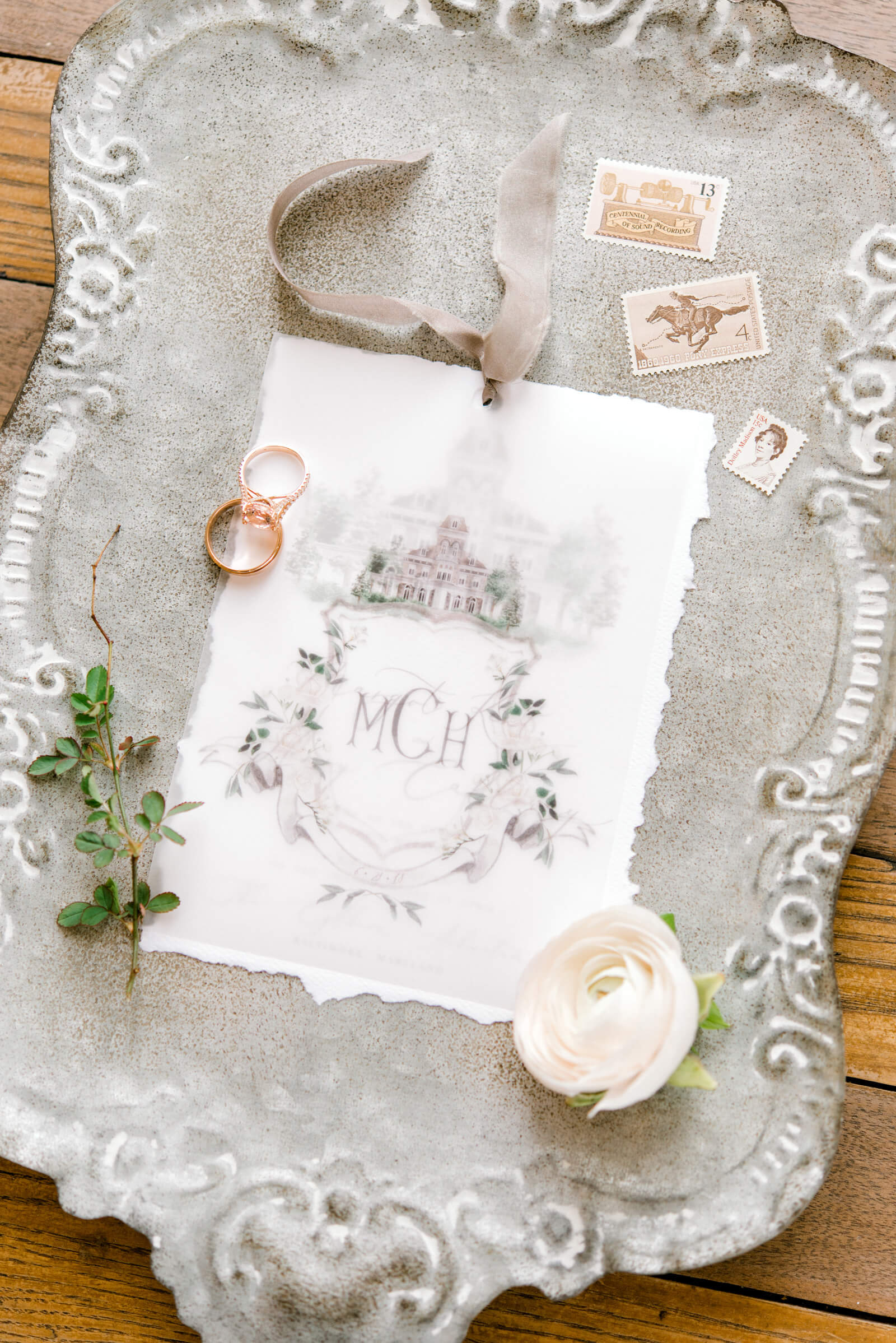The image depicts a grainy, ornate, rectangular tray that resembles a silver platter but has a textured appearance akin to rock. Positioned on a wooden surface with visible slats, the tray features intricate floral designs on its trim, especially prominent on the top and bottom edges. Central to the platter is a large, torn-edged card of what seems to be a wedding invitation or commemorative page, adorned with an illustration of a grand estate, the letters "MCH" framed in a wreath of leaves. A ribbon tied at the top of the card is also visible. On the lower right corner of the tray lies a white rosebud, while the lower left corner holds a sprig of green leaves. Scattered around the tray are three antique stamps: one depicting a horse with a 4-cent denomination, another showing a Morse code machine labeled 13 cents, and a smaller stamp featuring a woman's portrait. On the left side of the card, atop one another, rest two rings—a gold band and a silver band with a diamond, symbolizing a union. The detailed arrangement of the items suggests a theme tied to an elegant, perhaps vintage, wedding ceremony.